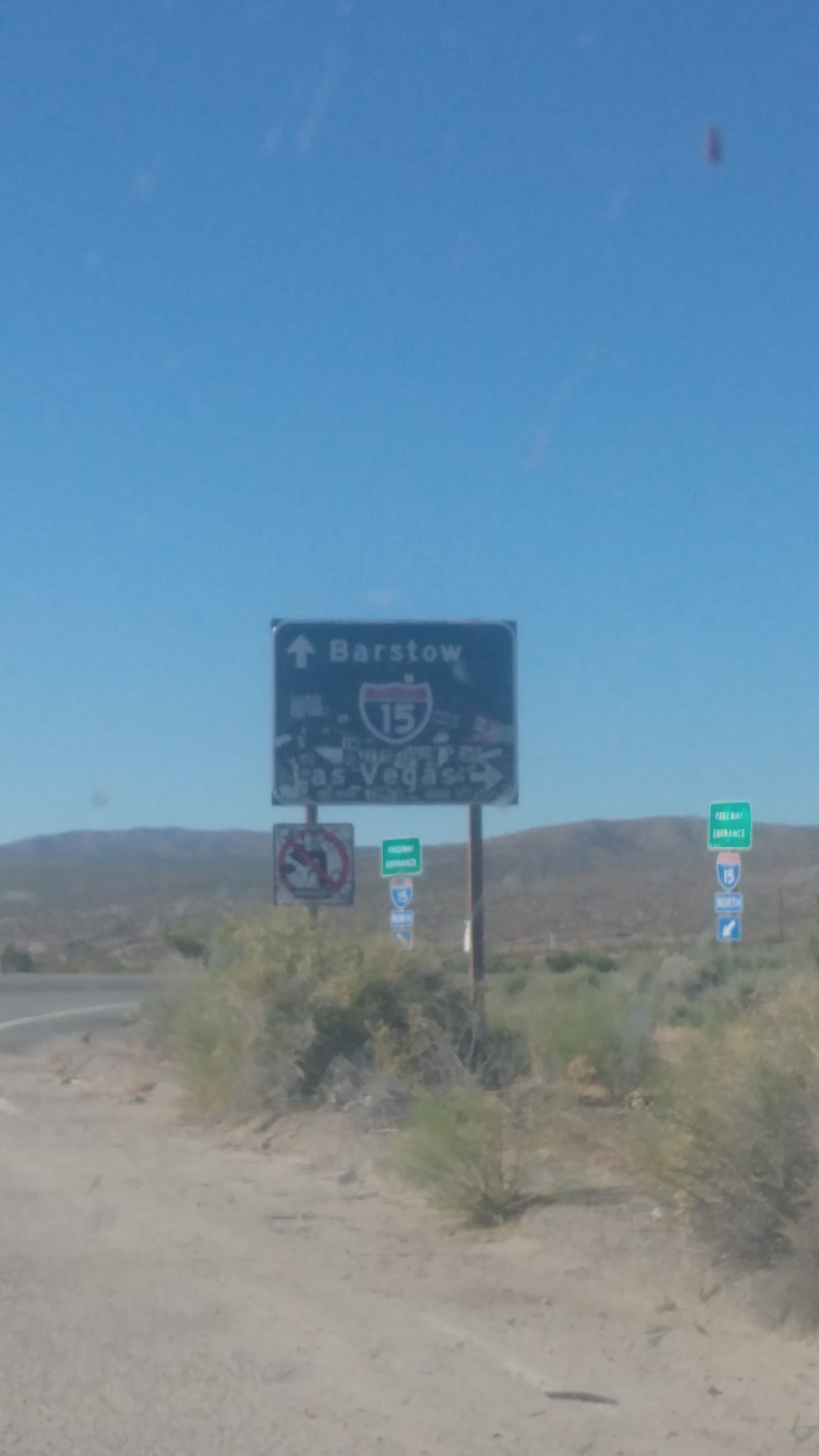This photograph captures a highway sign positioned along a desolate, desert highway. The central focus of the image is a large, green rectangular sign elevated on two wooden posts, directing travelers to their destinations. At the top of the sign, the word "Barstow" is prominently displayed, accompanied by an upward-pointing arrow. Below that, the word "Las Vegas" appears with an arrow indicating a right turn. In the middle of the sign, a shield-like emblem showcases the number "15," indicating the highway route. Additional signs can be seen nearby: one for the on-ramp and another that reads "No Left Turn." The surrounding landscape is characterized by arid, sandy earth and sparse, dry vegetation, emphasizing the barren nature of the area.